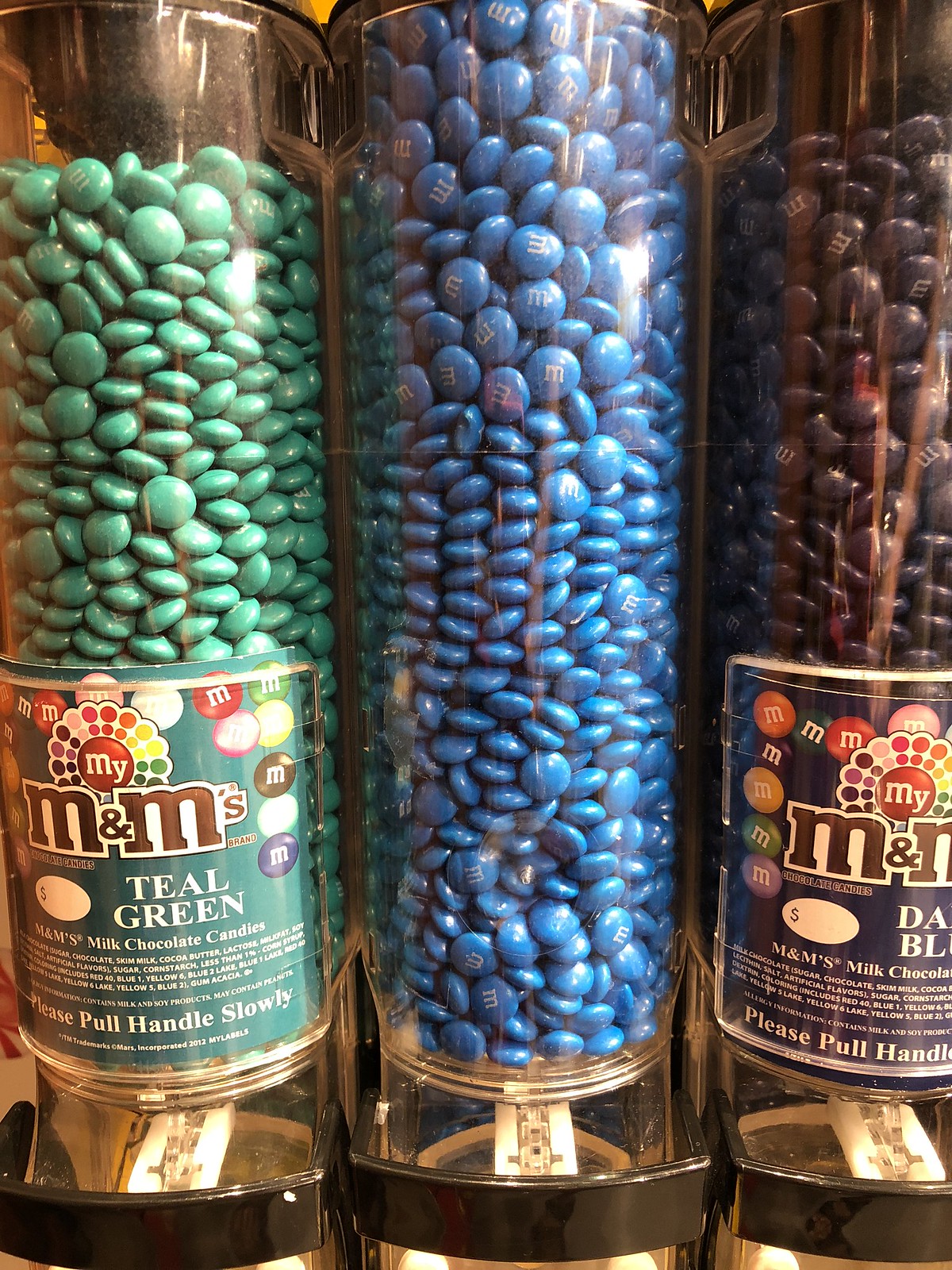This close-up image features three long cylindrical containers made of clear plastic, typically found in candy stores, possibly even at the M&M store in Las Vegas. The cylinders are filled with M&Ms in different colors and are equipped with black plastic levers at the bottom, which dispense the candies when pulled slowly. 

The left container holds teal green M&Ms, clearly labeled "teal green" with additional text reading "M&M smooth chocolate candies." The middle cylinder is filled with traditional blue M&Ms, but lacks a visible label. The rightmost container contains dark M&Ms, with a partially visible label that seems to read "dark blue" or "dark black," though parts of the words are cut off.